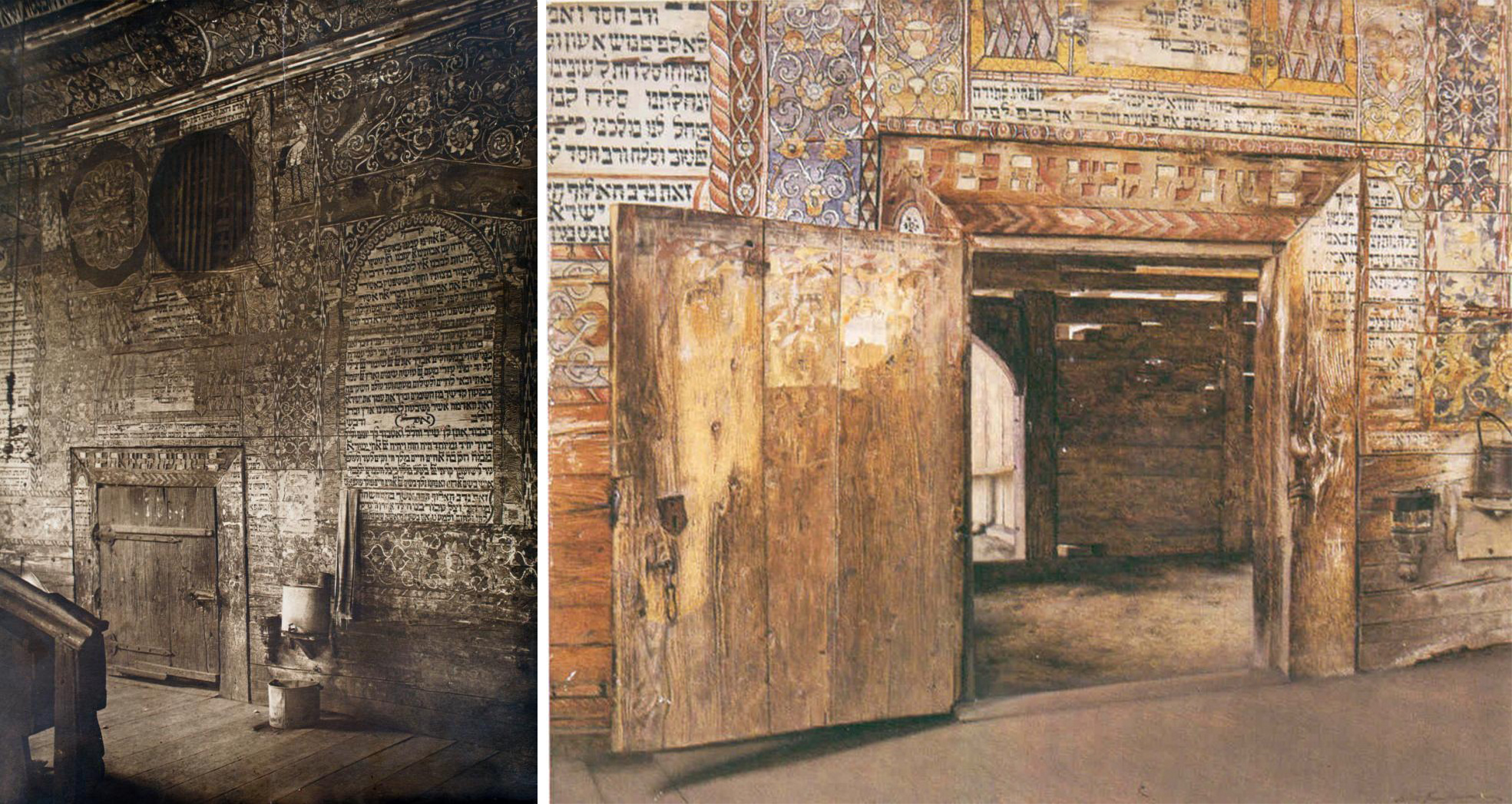The image features a black and white collage art divided into two sections. On the left side, there's a monochrome photograph of a large brick wall adorned with various arc-shaped designs and written text. The top-left corner of the wall features two circles, one containing vertical lines and the other intricate designs. Below the wall, there is a wooden door and a hardwood floor. The right side of the image appears to be a close-up, more detailed depiction of the same scene, possibly in the form of a painting. This part of the collage shows the wooden door swinging open, revealing additional text, which seems to be in Hebrew, and a similar arc-shaped wall design. The floor in this section of the image is portrayed in a grey color, accentuating the overall monochromatic and detailed artistic theme.